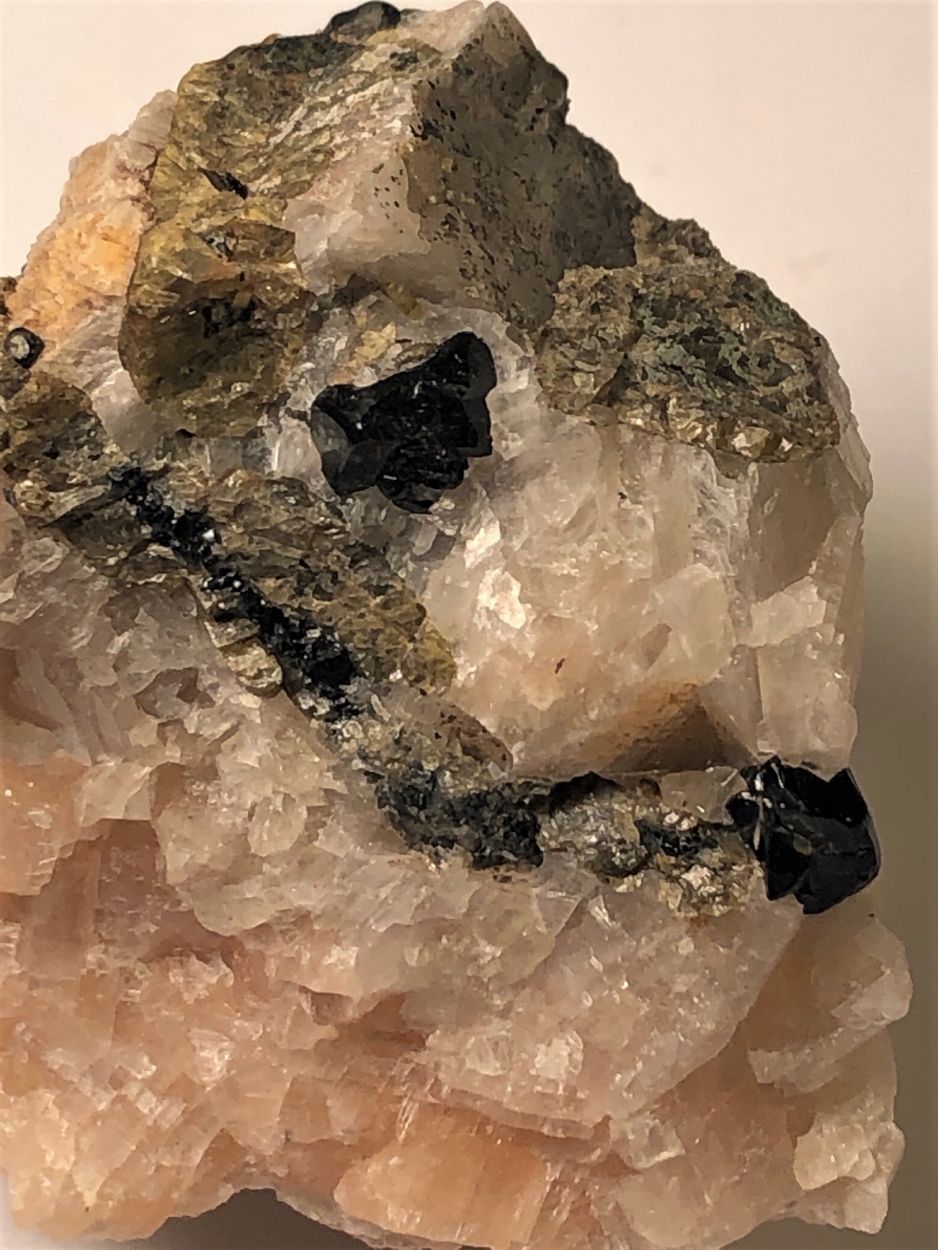The photograph showcases an extremely close-up, macro view of a jagged, multi-colored rock or mineral, potentially resembling a geode. Dominating the composition, the rock is centrally positioned but leans slightly towards the bottom left. The detailed texture is emphasized, revealing a rough, jagged surface that would feel coarse to the touch. The coloration of the rock is layered, starting with pink hues at the bottom, transitioning to a creamy white, then featuring a thin black line in the middle. Above this line, the pattern alternates between pink and white again, interspersed with black speckles and culminating in a greyish top layer. The overall shape of the rock is kind of square with a pointed top, set against a light brown or peachy background, likely a wall, with shadows cast to its right. No text is present in the image, allowing the intricate details and varied colors—ranging from tan, brown, gold, black, white, to pink—to be the focus.